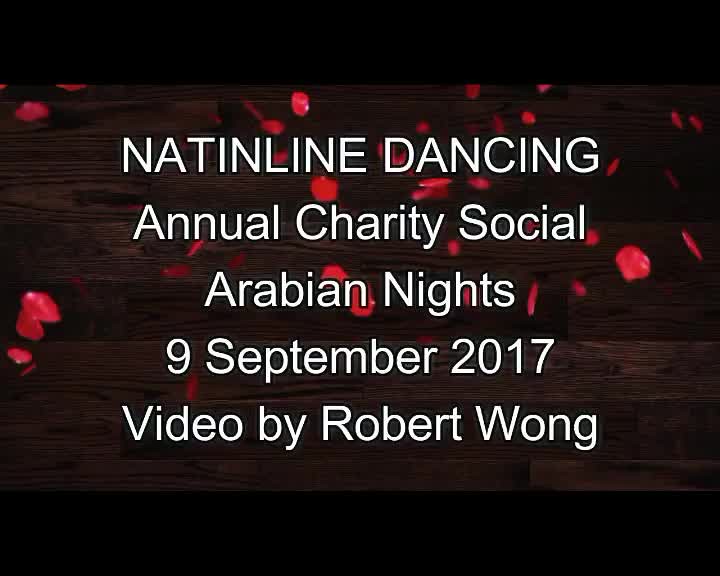Announcement: PowerPoint Slide or Website Visual

The image is a captivating announcement with a background resembling a dark wood grain surface adorned with scattered rose petals. Dominating this aesthetically pleasing design are splashes of red—ranging from dark and deep shades to bright accents. The text, prominently displayed in white, contrasts sharply against this dramatic backdrop.

At the top, in all capitals and larger font, it reads: "NET INLINE DANCING". Below this, in a slightly smaller and more uniformly structured font, the words "Annual Charity Social" appear, with each initial capitalized. The subsequent lines follow a descending size hierarchy, maintaining a harmonious arrangement:

- "Arabian Nights"
- "9th of September 2017"
- "Video by Robert Wong"

The overall appearance suggests this graphic is an opening slide for a video, specifically designed to advertise the Net Inline Dancing Annual Charity Social event themed "Arabian Nights." The simplicity and elegance of the design indicate its use in digital platforms such as PowerPoint presentations, websites, or social media posts.